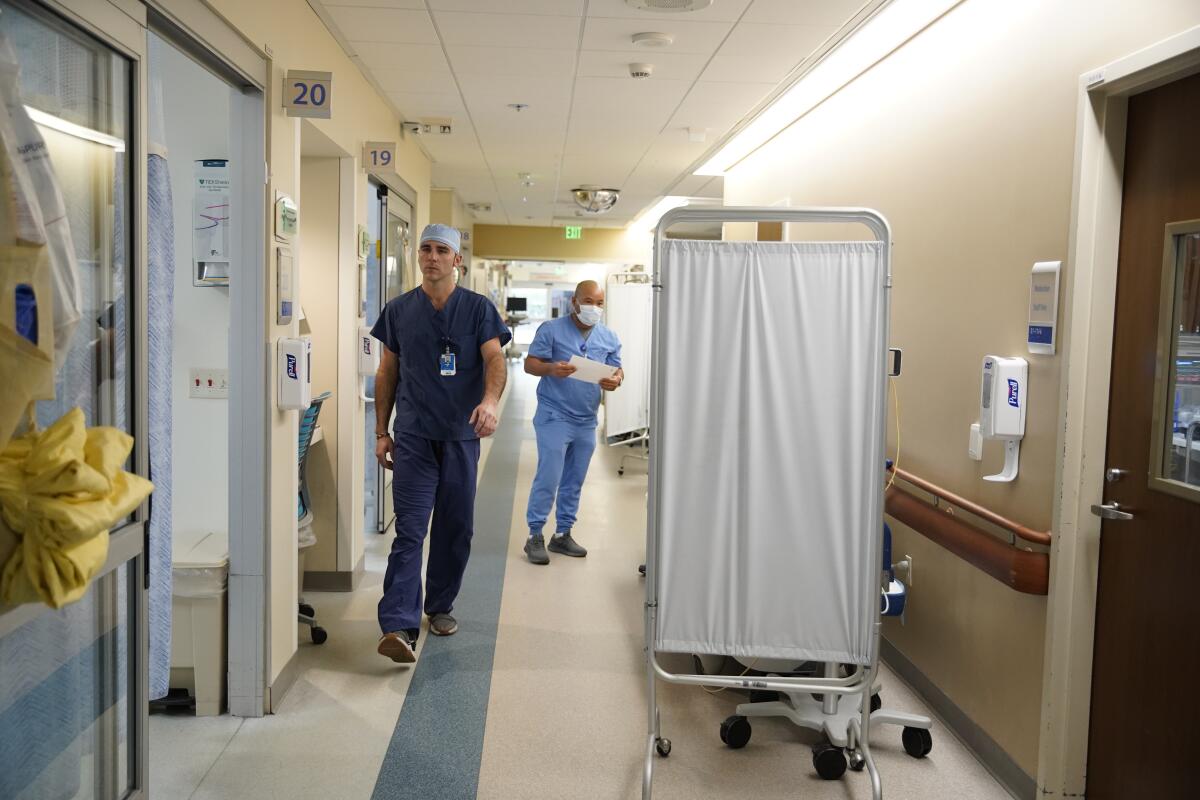The image portrays a bustling corridor in a hospital, potentially an ER or surgery center, with rooms closely spaced on either side, numbered 19 and 20. The white-tiled floor features a distinctive long blue strap running through the hallway. On the walls, typical hospital fixtures can be seen, including multiple Purell hand sanitizer dispensers, protective gear, and a screen that could be used for patient privacy. 

In the background, a healthcare professional in light blue scrubs and a face mask is holding a chart and possibly reading from it. Moving towards the camera in the foreground is another staff member in navy blue scrubs and a surgical cap, mid-step with his right foot poised to touch the ground and arms swinging naturally. The corridor also showcases open doors with curtains on the left side, a closed wooden door on the right, an exit sign, and standard rolling computers used for patient information and administrative tasks.